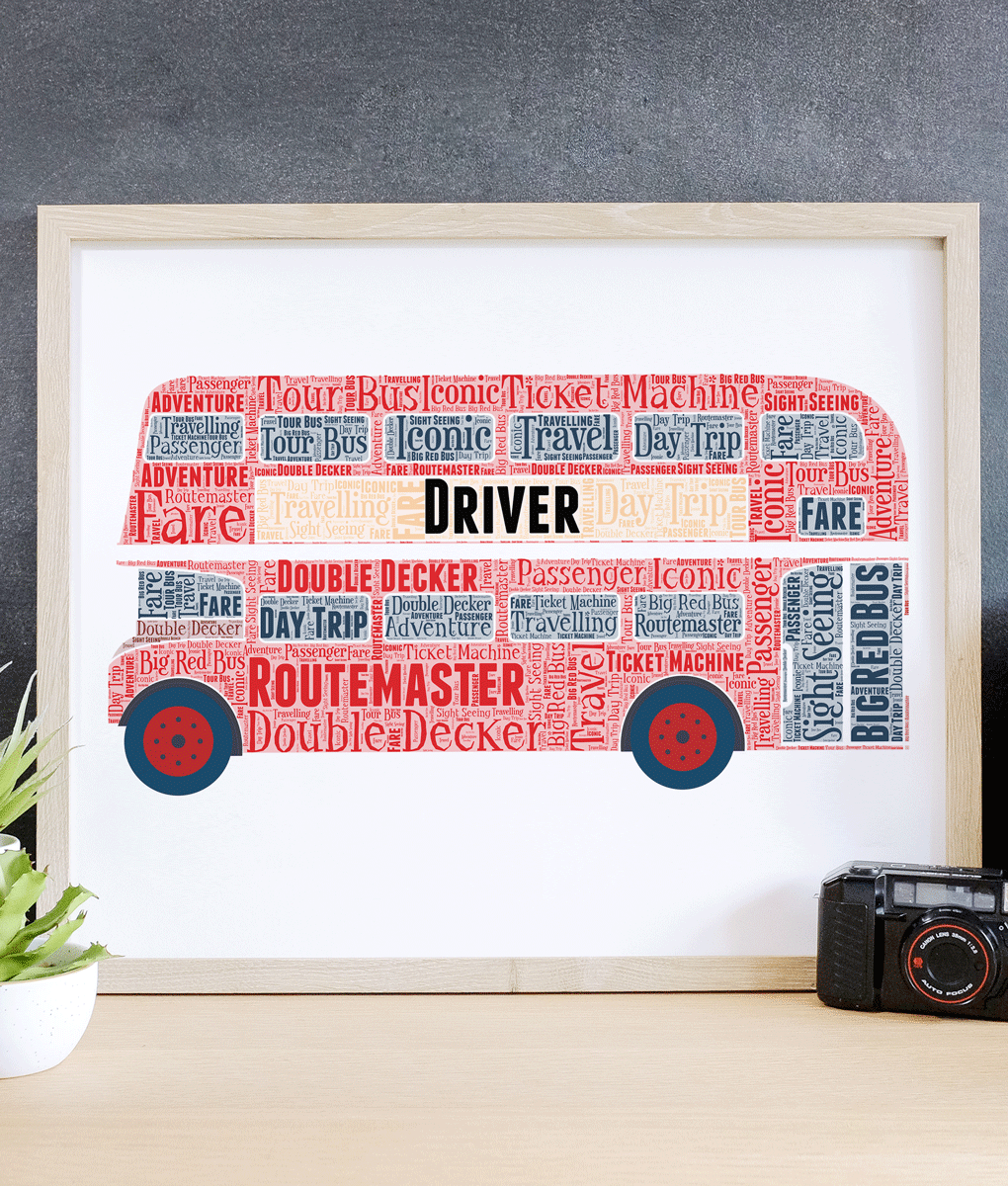The photograph captures a framed artistic piece featuring a red double-decker bus made up entirely of words. The image is vertically rectangular and prominently staged indoors with artificial lighting. The frame surrounding the artwork is light beige with no specific border, and the background is white, emphasizing the vivid red of the bus. The bus is shown in profile, with the front facing the left side of the image. It has black tires with red rims, and the upper part includes a yellow section labeled "DRIVER" in black text. The artwork's creative use of text to form the bus and its details contributes to its visual appeal. The bus appears to be a London sightseeing tour bus, suggested by its detailed and repetitive use of words like "roadmaster," "ticket machine," and "tour bus." The framed piece rests on a brown desk or countertop, with a small white planter holding a green plant in the lower-left corner and a vintage-style black digital camera in the lower-right corner. The backdrop is a dark blue or black wall, contributing to the focused and curated presentation of the scene.